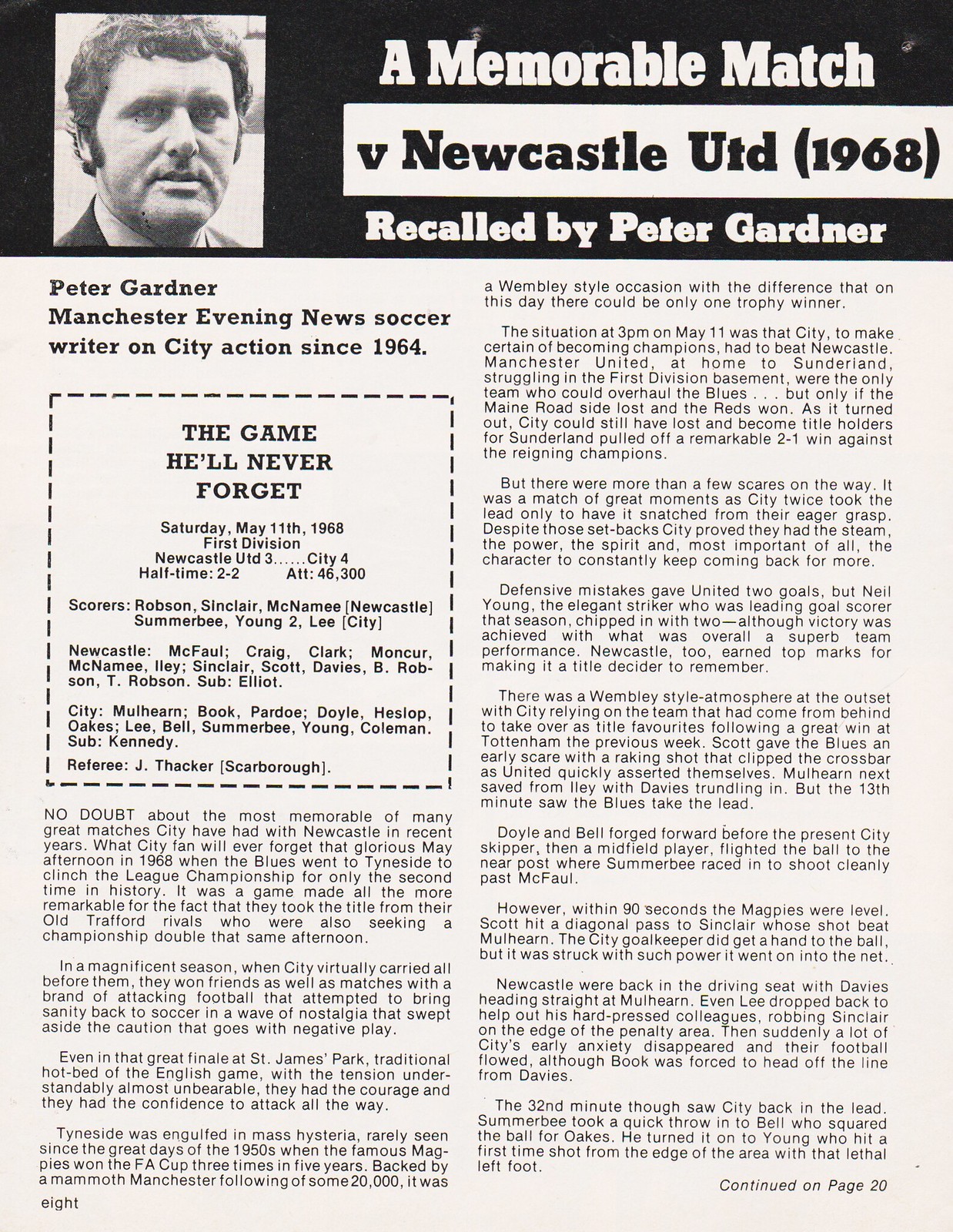The image is a black-and-white page from an old magazine or newspaper, presumably from the Manchester Evening News. At the top of the page is a black strip featuring a photograph of Peter Gardner on the left side. The headline on the right reads "A Memorable Match Versus Newcastle UTD 1968, Recalled by Peter Gardner," indicating that Gardner is both the subject and the author, who has been a soccer writer covering City Action since 1964. Below this, a prominent boxed section is titled "The Game He'll Never Forget," detailing a First Division match that took place on Saturday, May 11th, 1968, where Newcastle Utd played against City, ending with a 4-3 score in City's favor after a halftime tie of 2-2. The box also lists players, scorers, and the referee. The main article is divided into two columns detailing Gardner's recollection of the memorable match, with instructions at the bottom right to continue reading on page 20.